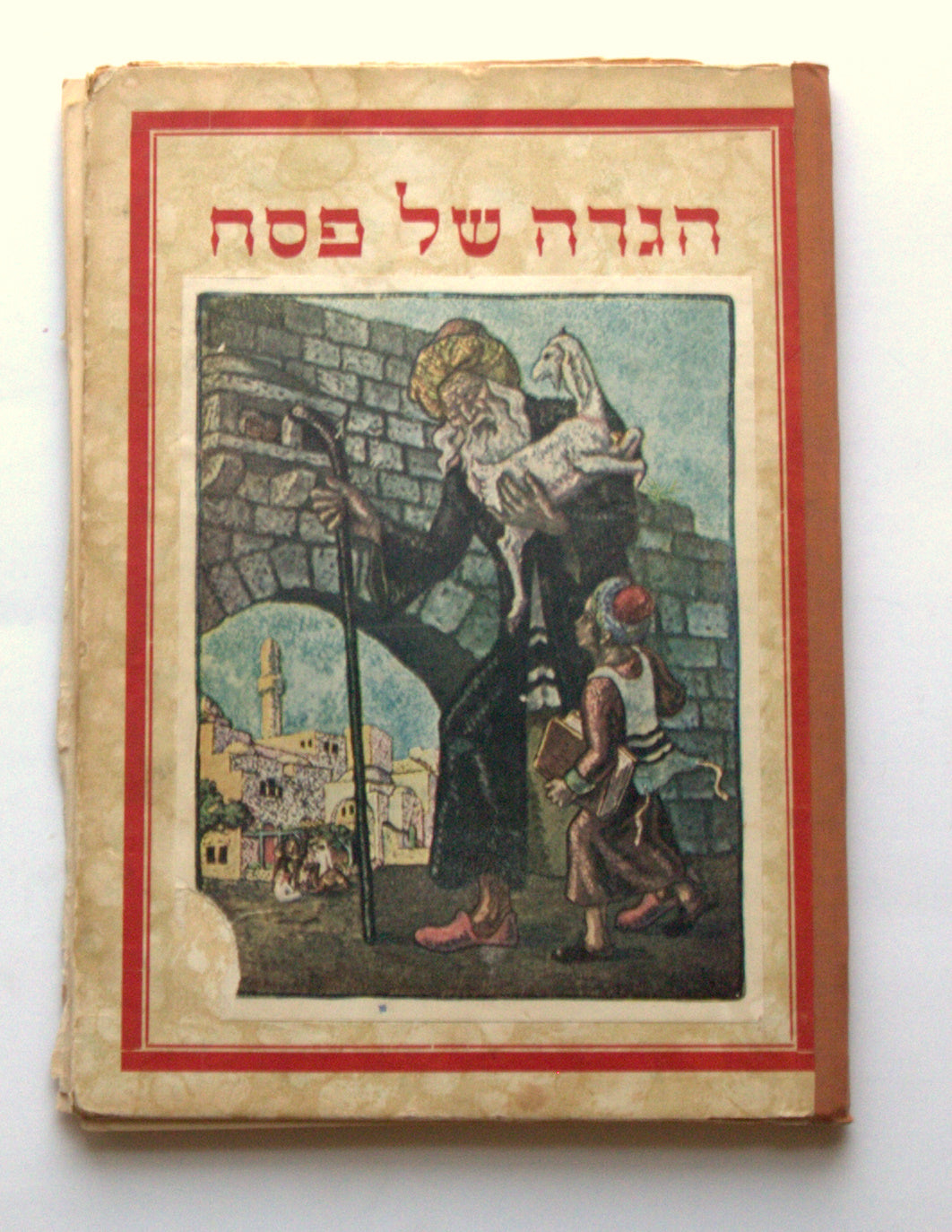This image is the back cover of an old, possibly water-damaged school children's textbook, encased in a red border. The cover features an intricate illustration set against a white background. Central to the illustration is an elderly man, who appears to be a shepherd, dressed in a black robed cloak and a robed headdress. He has a white beard and is adorned with red penny loafers. In his left hand, he holds a goat while leaning on a walking stick with his right. To the bottom right, a young boy, clad in a red robe and hooded hat with black penny loafers, gazes up at the shepherd for guidance, clutching a large school book. The scene unfolds in what seems to be an ancient city, with a stone cobbled archway entrance on the left which opens into a town. Behind them, the blue sky peeks through, adding a touch of serenity to the backdrop. Above the image, there is an inscription in Hebrew, likely referencing a Passover legend, as the book is old and appears to tell a story related to this tradition. The spine of the book shows signs of age, possibly reinforced with brown tape, indicating its historical value of possibly over a hundred years.